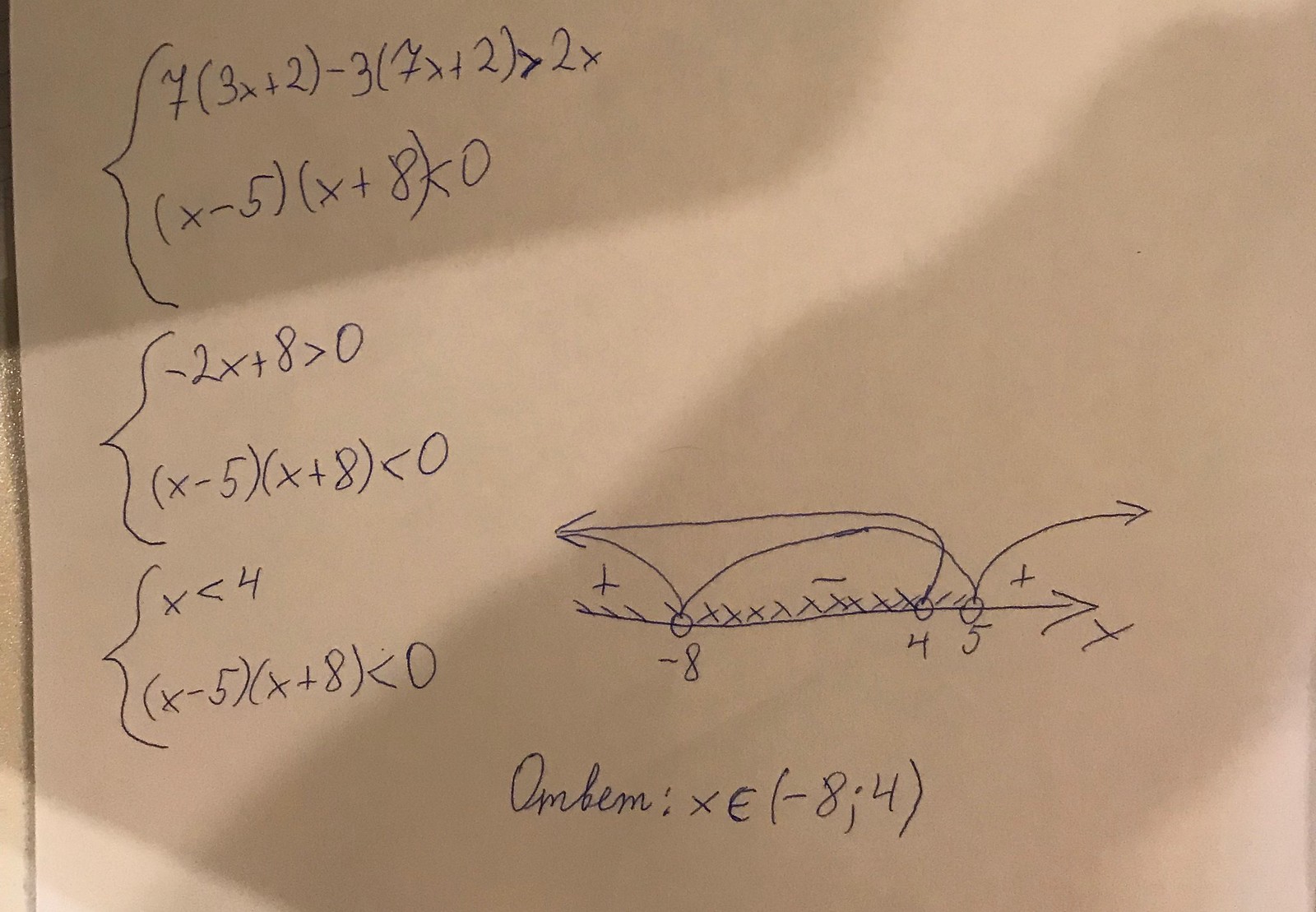The image shows a sheet of tan-colored paper featuring handwritten mathematical equations and graphs in blue ink. The top left section of the paper contains a series of inequality problems. The first line reads:

\[ 7(3x + 2) - 3(7x + 2) > 2x \]

Below it, there is another equation:

\[ (x - 5)(x + 8) < 0 \]

Both equations are connected by annotations, indicating their relation. Another inequality, positioned beneath the previous one, states:

\[ -2x + 8 > 0 \]

This is followed by a repetition of the earlier equation:

\[ (x - 5)(x + 8) < 0 \]

Continuing down the left-hand side, the equations persist with variations:

\[ x < 4 \]
\[ (x - 5)(x + 8) < 0 \]

To the right of these equations, a graph has been sketched. This graph includes an axis line pointing horizontally, with marked points at \(-8\), \(4\), and \(5\). Small "x" marks are plotted along the axis between these numbers. Connecting lines and arrows illustrate relationships between these points.

At the bottom of the page, in cursive handwriting, there is a note reading:

\[ \text{ombem:} \ x \ \epsilon \ (-8; 4) \]

This complex array of mathematical notations and relationships appears to outline a detailed series of steps for solving inequalities, supplemented by a corresponding graph to visualize the solution set.